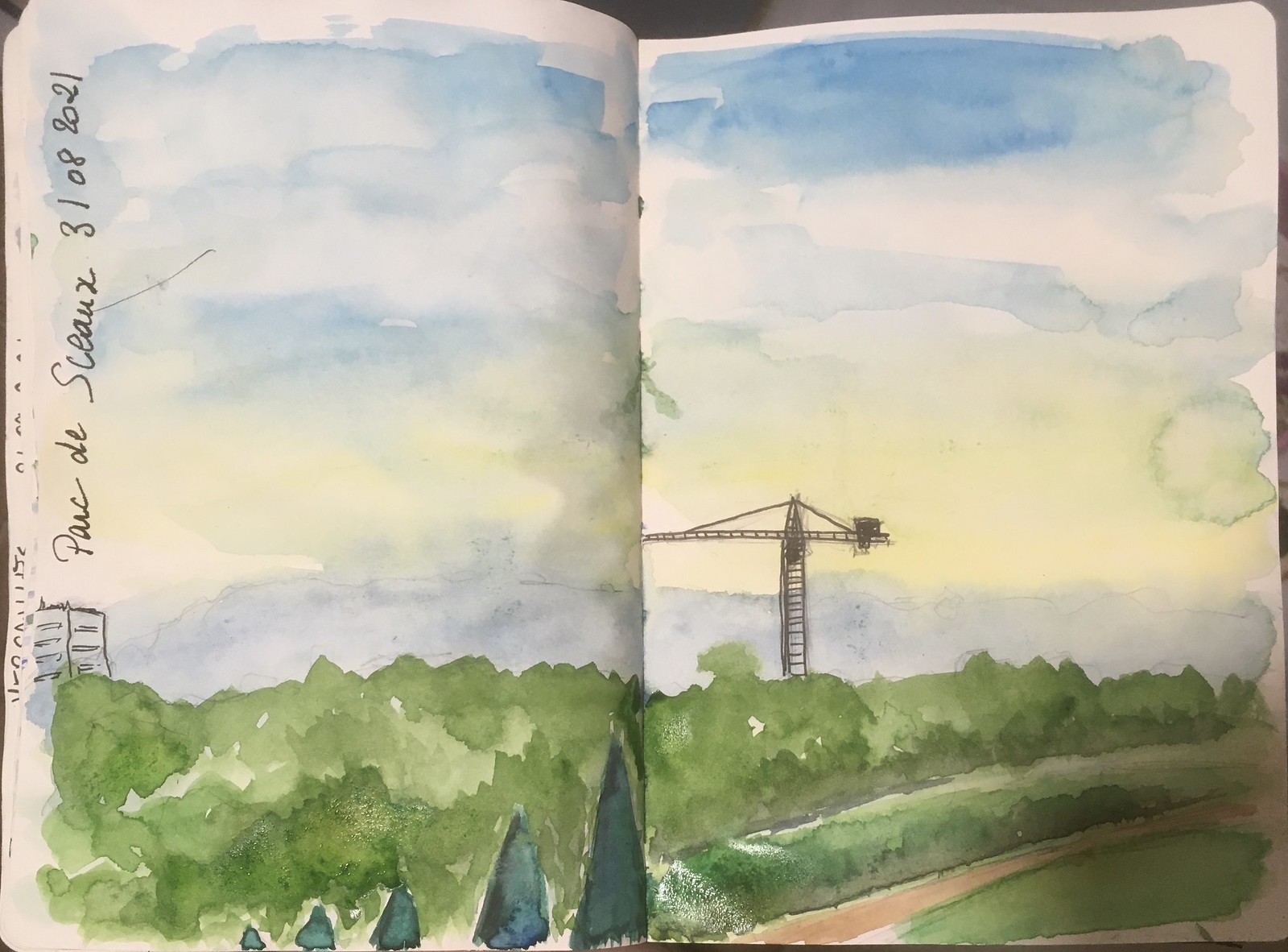In the picture, an open book is displayed, revealing a watercolor painting that spans both pages. The binding runs down the middle, clearly identifying it as part of a collection of watercolor sheets. The artwork depicts a lush, green scene featuring various sizes of dark green pine trees and bushes stretching across from left to right. Prominently, there is a brown dirt path leading through the green field, with another path seen at the lower right section of the painting. The vibrant blue sky above is clear and unclouded, creating a tranquil backdrop. Notably, a crane extends upwards in the distance, suggesting construction, yet no construction sites are visible nearby. On the far left above the tree line, an apartment or office building can be seen. Additionally, a drip mark stains the painting, indicating a spill. Along the edge of the picture, text in black ink reads "Parc de Sion X" spelled P-A-R-C-D-E-S-I-O-N-X S-C-E-A-N-X, followed by the date 31.08.2021.